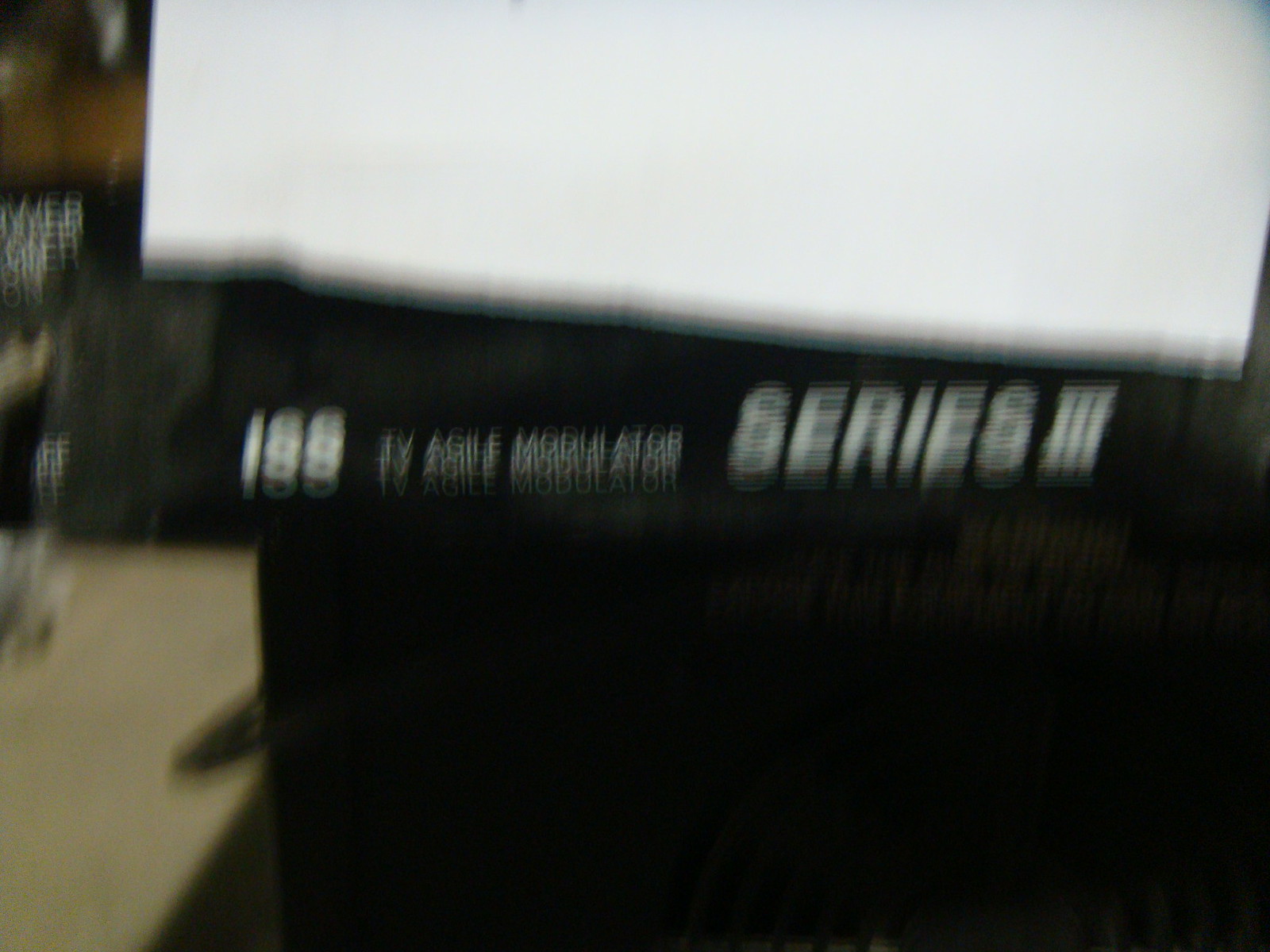The image appears to be a blurry, real-life photograph capturing a piece of equipment. Dominating a significant portion of the image is a black device with a black bar that features white text. The text reads, "I ISS TV Agile Modulator Series III." Above this text area, there's a rectangular white section, possibly a piece of paper or a label, partially hanging down but cut off by the top edge of the image. To the left of the device, in the background, there seems to be a light wooden table surface with an indistinct skinny object resting on it. The overall image quality is poor, with noticeable blurriness and graininess, as if taken without proper focus or while the camera was moving.